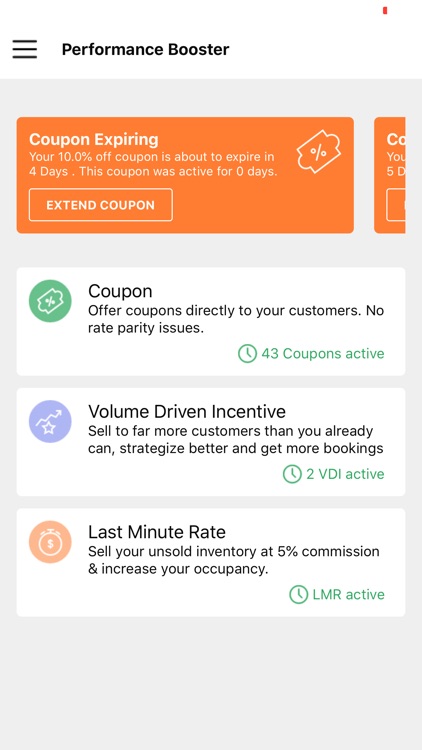The image depicts a mobile application interface designed for managing promotional coupons and incentives. The top section features a white background with a three-line pullout menu icon on the left. The title "Performance Booster" is prominently displayed in black text.

Below the white header, the rest of the page transitions into a light gray background. The main content is organized into several rectangular sections. The first rectangle, highlighted in orange, provides information about an expiring coupon: "Your 10% off coupon is about to expire in four days." It notes the coupon's 40-day activity period and includes an orange button with the text "Extend Coupon" in white.

Following this, another section with a white background features a green circle, accompanied by the text "Coupon Offer: Coupons directly to your customer, no third-party issues. 43 coupons active," displayed in green.

Next, a section with a blue circle offers volume-driven incentives: "Sell to far more customers than you already can strategize better and get more bookings," alongside a clock icon indicating "2 Active" in green.

The final section displays an orange circle with the last-minute rate promotion: "Sell your unsold inventory at 5% commission and increase your occupancy."

Each section is color-coded and uses clear, concise text with actionable buttons to guide the user through various promotional strategies and coupon management tools.